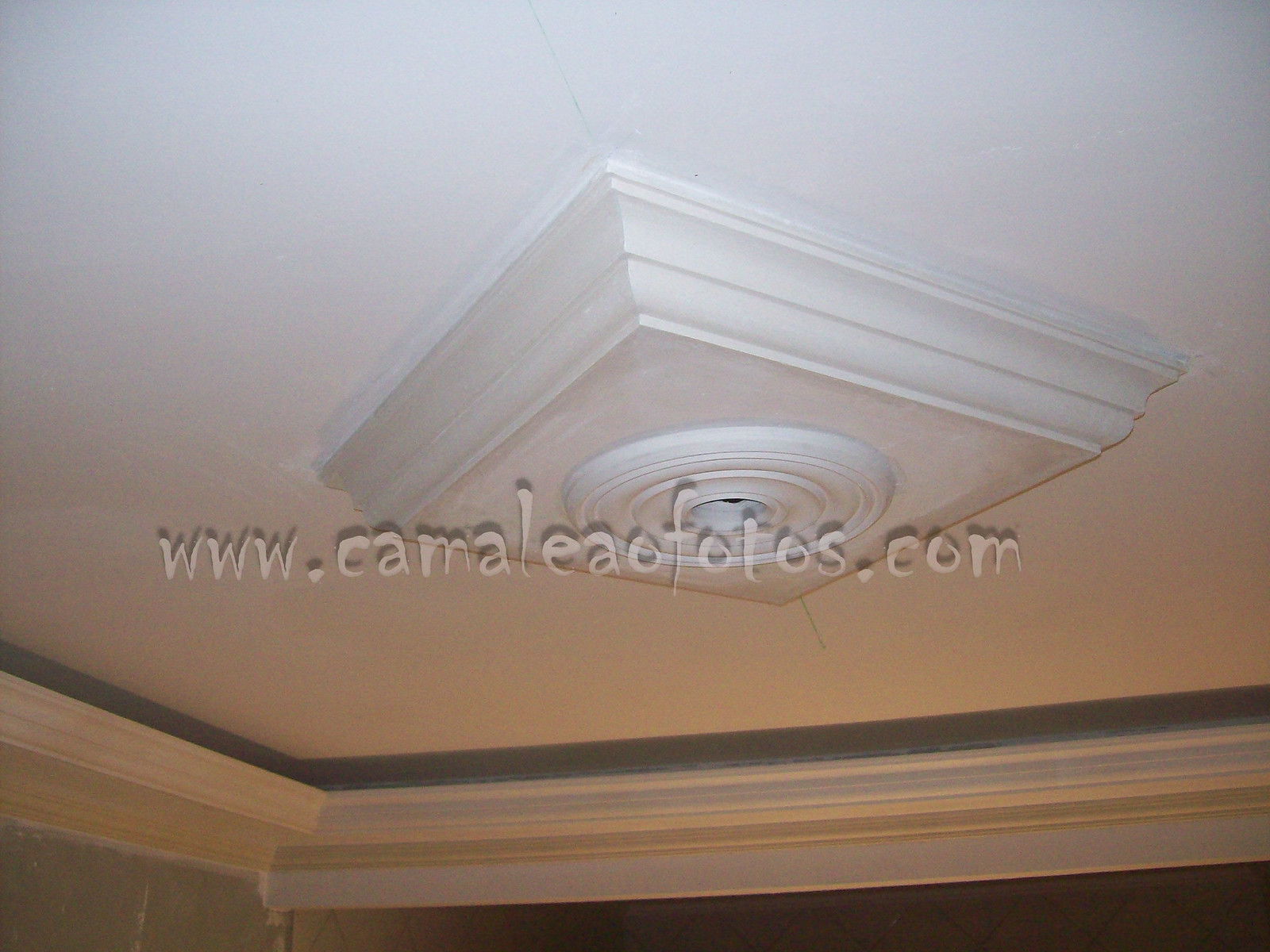The image, likely intended for an advertisement, prominently features a tray ceiling in a room with white trim and a slightly darker beige or grayish wall. The ceiling, also white, showcases a two-level lighting fixture area that is flush within the structure but extends out slightly. This area is painted a deeper shade of white. At the center of this fixture is a round circle with an empty socket, suggesting a place for a lightbulb or possibly a hidden camera. Surrounding this focal point, the ceiling is bordered by white trim, creating a distinct separation from the walls. The room is dimly lit, with a soft light source brightening the lower portion of the image. Centered below this setup, in white letters with shadow effects and a slightly eerie font, is the website: www.CAMALEAOFOTOS.com.